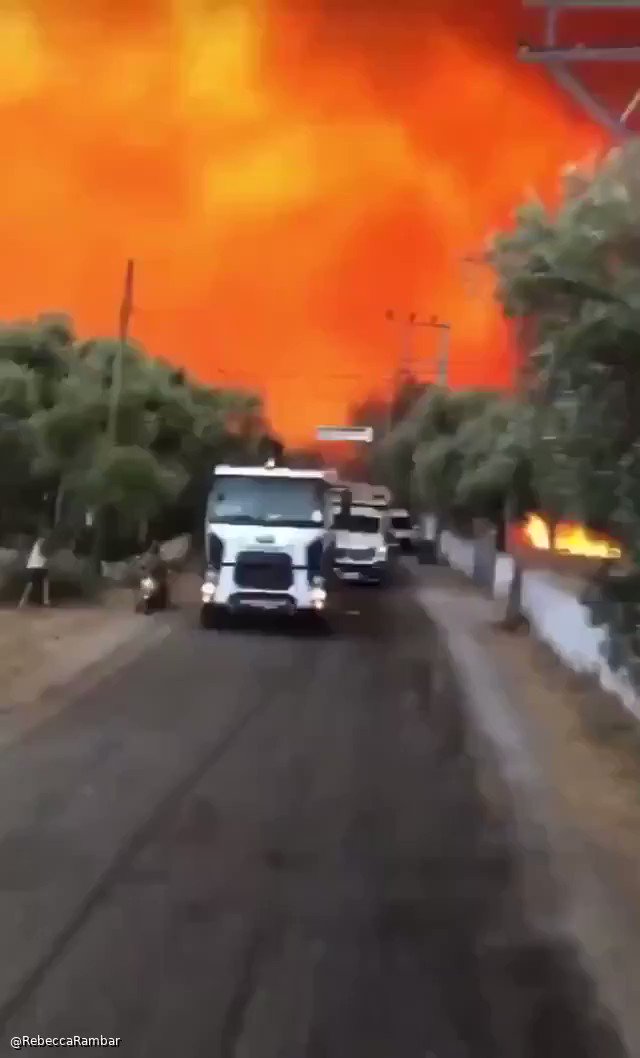This color photograph captures a dramatic scene of two white trucks with black accents driving on a dark gray asphalt road towards the camera. The road is bordered by light gray-brown sidewalks and low white fences or walls on either side. The street is flanked by lush green round trees. To the right of the image, a smaller fire can be seen behind the white fences. In the background, a massive, vibrant orange blaze dominates the sky, creating a stark contrast with the surrounding greenery and filling the top third of the frame, suggesting a dire emergency situation. Additionally, there are telephone poles visible in the backdrop. A person is walking on the sidewalk to the left, and at the bottom left corner of the photo, white text reads "@RebeccaRambar." The overall setting of the photograph is outdoors, with a clear vertical orientation. The vivid colors include shades of red, orange, yellow, brown, dark green, white, black, gray, and beige, adding to the urgency and intensity of the scene.